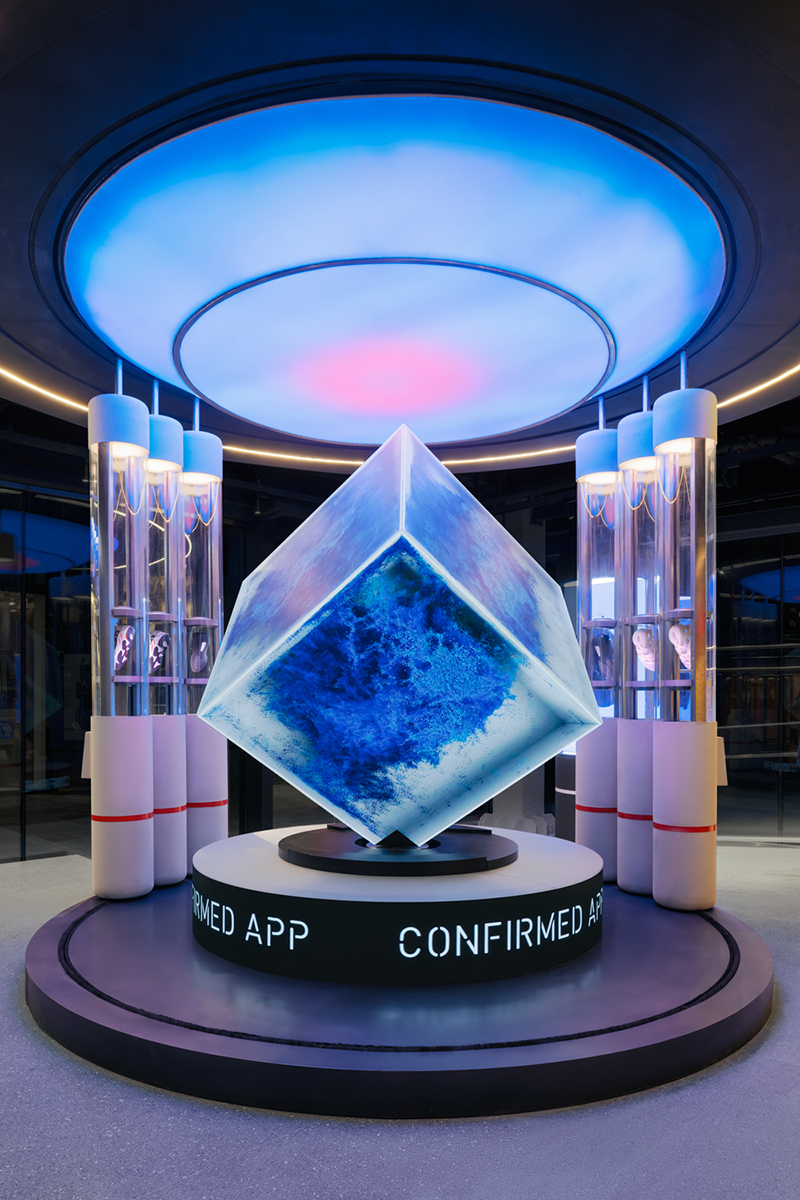The image depicts a futuristic exhibit, possibly in a space museum, featuring a striking digital art piece at its center. A transparent cube, floating diagonally, contains dispersed blue dye that gives it a cosmic, icy appearance. The cube is mounted on a black, round pedestal labeled "Confirmed App" in white lettering. Surrounding the pedestal are several large, scientific test tubes, six in total—three on each side. Each tube has white bases and caps, with clear sections displaying intricate red and blue wires within. Above the display, a prominent bluish dome light casts a cool, ethereal glow over the scene, with a subtle accent of pink light emanating centrally. The background remains dark, adding to the enigmatic, cosmic ambiance of the exhibit.